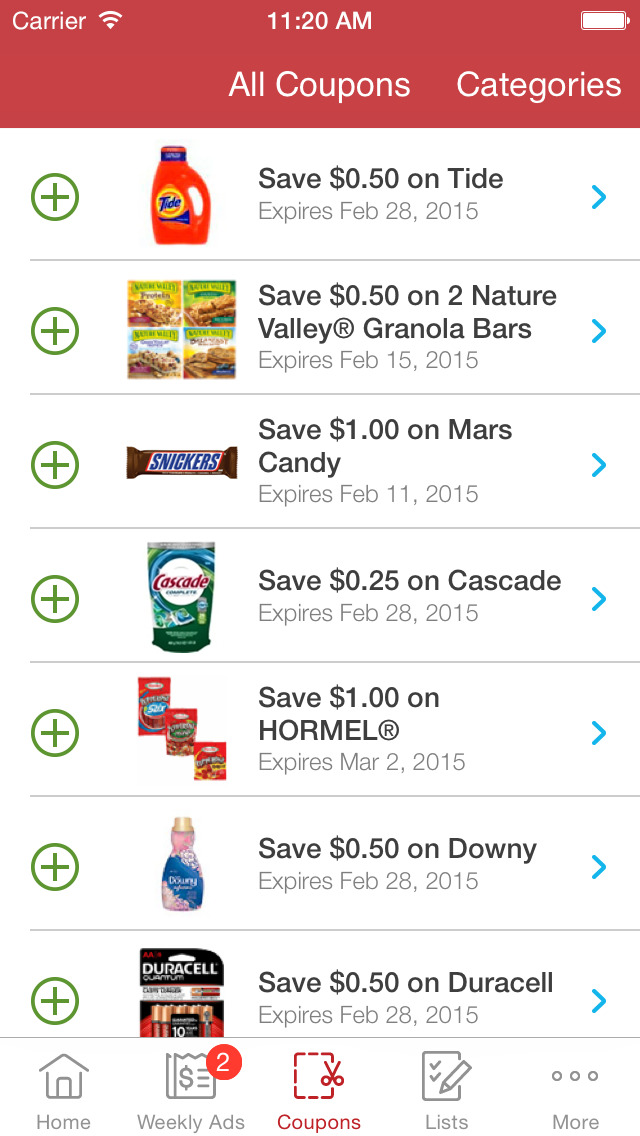This detailed screenshot from a coupon app provides an organized and comprehensive overview of various discount offers and menu options available to users. 

At the very top, a red banner displays crucial mobile phone status indicators: carrier signal strength, a full Wi-Fi signal, the time (11:20 a.m.), and a full battery icon. Directly beneath this, still within the red rectangle, are the navigation options labeled "Coupons" and "Categories."

Below the banner, seven products are showcased, each separated by a thin gray line to ensure clarity. On the left-hand side of each product listing is a green circle with a plus sign, allowing users to expand for more details. Each product includes a photograph, a savings amount, and an expiration date:

1. **Tide Washing Liquid:** Save $0.50; expires February 28, 2015.
2. **Nature Valley Granola Bars:** Save $0.50 on two packs; expires February 15, 2015.
3. **Snickers (Mars Candy):** Save $1.00; expires February 11, 2015.
4. **Cascade Dishwasher Tablets:** Save $0.25; expires February 28, 2015.
5. **Hormel Product:** Save $1.00; expires March 2, 2015.
6. **Downy Fabric Conditioner:** Save $0.50; expires February 28, 2015.
7. **Duracell Batteries:** Save $0.50; expires February 28, 2015.

At the bottom of the screenshot, grey icons provide additional menu options: 

- **Home:** Represented by a small house.
- **Weekly Ads:** Symbolized by an icon resembling a newspaper with a dollar sign.
- **Notifications:** Indicated by a circle with the number two, signifying two new alerts.
- **Coupons:** Shown with a rectangle featuring a dotted line and scissors.
- **Lists:** Displayed with an icon of three lines.
- **More:** Indicated by three dots, offering further options.

This layout ensures users can easily navigate, select, and manage their desired coupons efficiently.